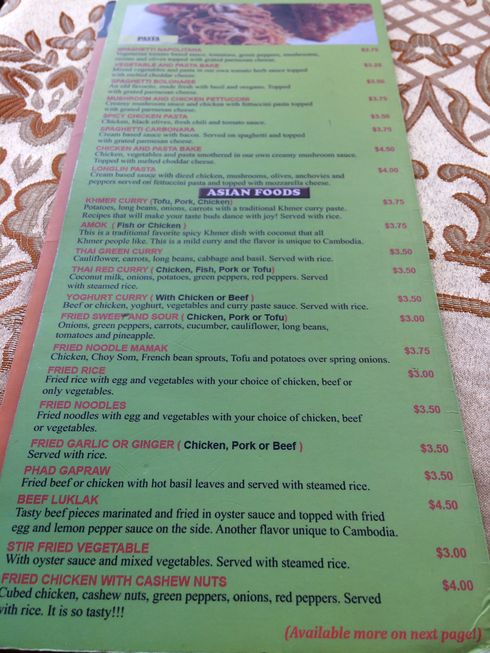This image displays a vertically-oriented, rectangular menu predominantly green in color, likely featuring an array of Asian dishes. The top portion of the menu showcases an image that appears to be a plate of spaghetti or a similar dish. The menu is placed on a table covered with a patterned cloth adorned with traditional motifs in white, dark brown, and greyish tones, including flowers and other designs.

The menu includes an orange left margin, with both the names of the dishes and the prices also presented in orange. The menu is divided into sections, with the top section seemingly dedicated to pasta dishes, where the highest price noted is $4. The section below offers a selection of Asian foods, with prices ranging from $3 to $4.50. The prices are aligned along the right margin, matching the orange color used for the dish names.